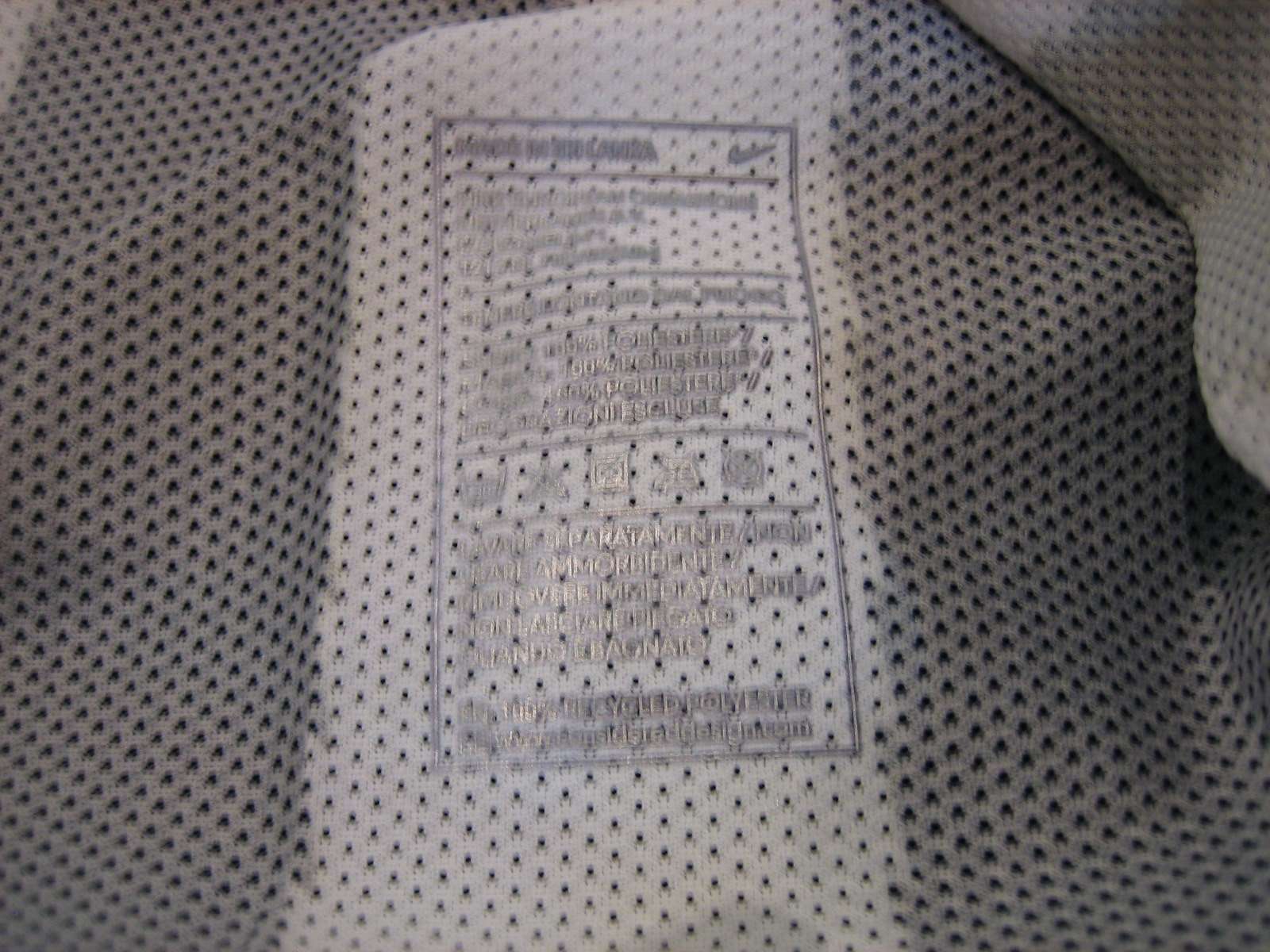This indoor photograph captures a close-up view of a printed care label on a perforated fabric, likely from a Nike athletic shirt. The fabric, which resembles breathable jersey material, features a pattern with vertical gray and white stripes. In the center of the image is a blurred white rectangle where a silver-inked label is printed, detailing the care instructions and displaying a noticeable silver Nike swoosh in the upper right corner. The fabric is predominantly light gray with folds and crumples, particularly evident in the top right corner, adding texture to the image. The perforations in the fabric reveal an underlying black layer, emphasizing the garment's breathable quality.